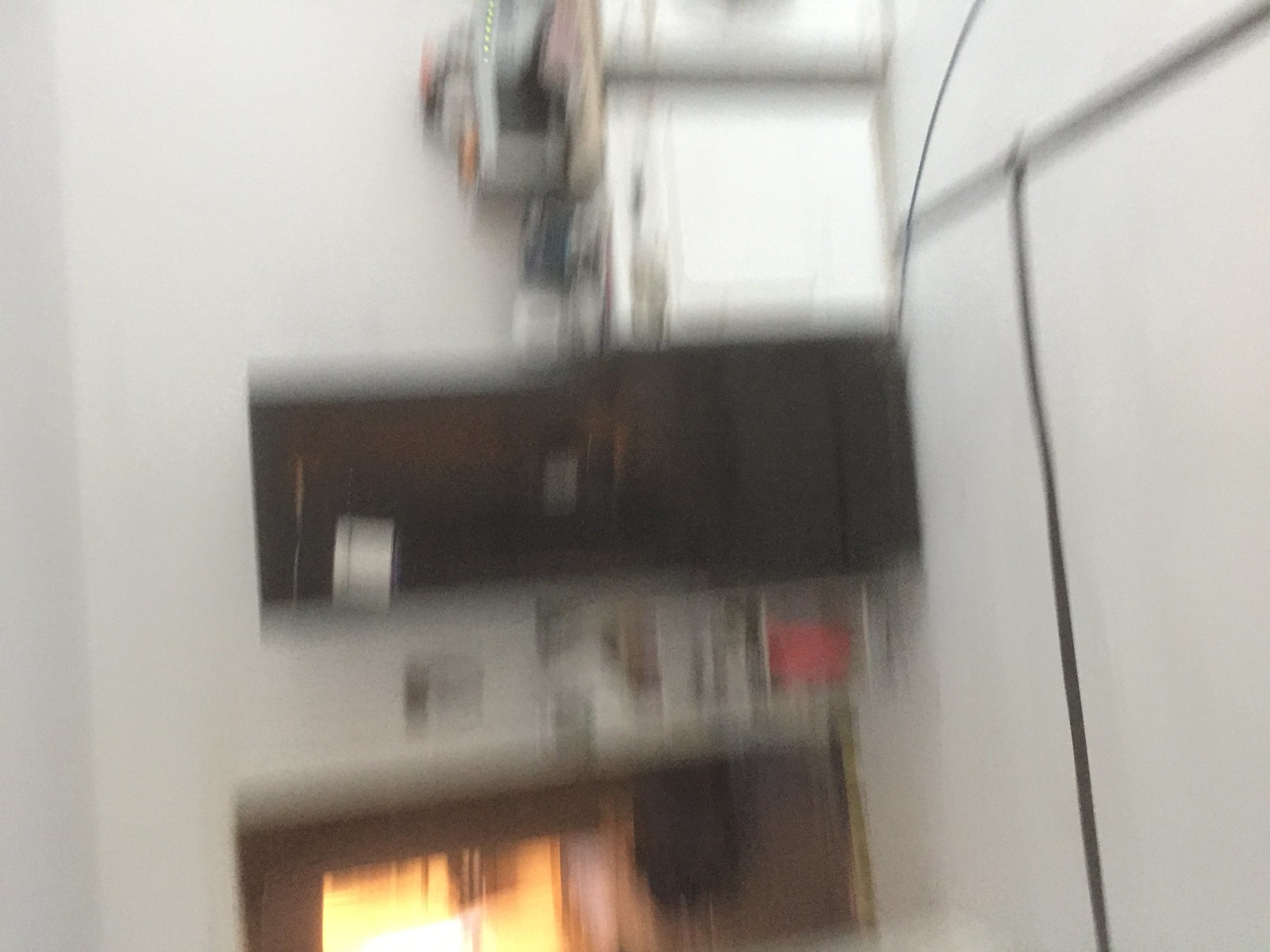The image depicts a disoriented, blurry interior scene, possibly of a house or office space. The picture is oriented on its side, with the floor visible to the right. A prominent black rectangular object appears in the center; though unclear, it might be a piece of office equipment or a doorway. Adjacent to it is a white, square structure, possibly cabinets, with various items placed on top. To the bottom left, there is an open doorway leading to another room, where a window is visible, allowing bright light to flood in. The floor features black stripes, and the wall behind the furnishings is white.